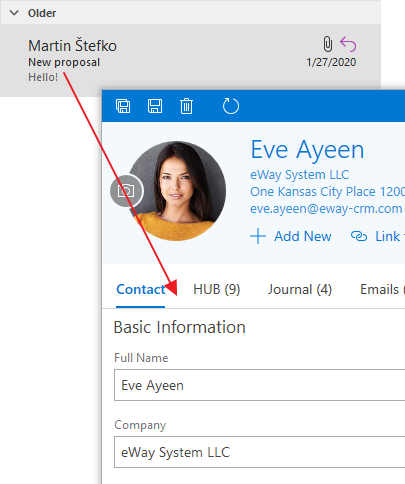This is a highly detailed screenshot from a webpage illustrating a user's profile and associated elements. At the top, there is a mid-gray bezel containing navigation text. On the left-hand side, there's a black arrow pointing to the word "Older". To the right, the name "Martin S. Té F.K.O." is displayed prominently in dark gray.

Beneath this header, the text "New Proposal" is shown, followed by a gray "Hello!" with an exclamation mark. On the right side, a black paperclip icon is accompanied by a curved purple arrow pointing towards it. Below this, a date is displayed: January 27th, 2020.

Central to the screenshot is a profile section featuring an image of a female with a dark gray background. She has black hair, light skin, an orange shirt, brown eyes, and pink lipstick, and is gazing towards the camera. Above her profile picture, a dark blue bezel includes icons for saving (two floppy disks), deleting (a trash can), and refreshing (a curved arrow pointing right).

To the right, blue text reads "Ava Aen Eve Ayeen", and below that, it says "E-Way Systems LLC, 1 Kansas City Place, Suite 1200". An email address is also provided: "Ava.Aeen@eway-crm.com". A section labeled "Add New" features a blue plus icon, and there are overlapping paperclips, indicating a link, which is partially cut off. A red arrow points downward from the "Older" section towards the profile.

The lower portion of the screenshot has navigational tabs— "Contact" is selected and underlined in blue. Other tabs include "Hub (9)", "Journal (4)", and a cut-off "Emails". Underneath, the basic information for the profile is displayed: "Full Name" is listed as "Ava Ayeen", and "Company" is listed as "E-Way Systems LLC".